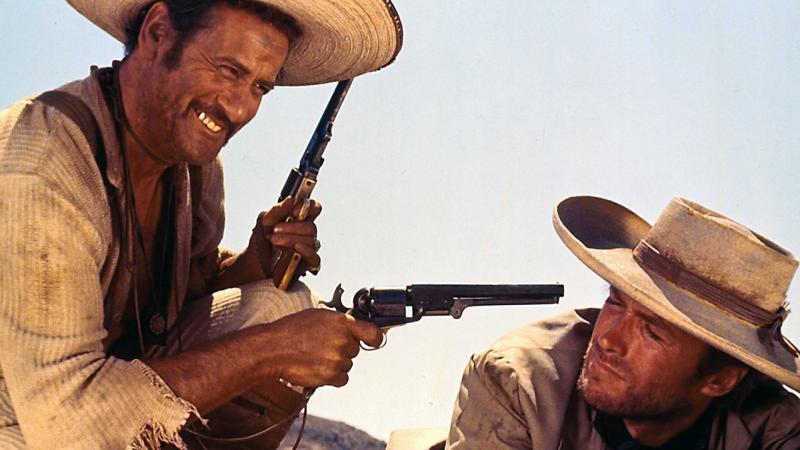The image is a detailed screenshot from an old western movie, possibly "The Good, the Bad, and the Ugly." It features two men prominently depicted in close-up. On the left side of the image stands a man with dark hair and tan skin, dressed in a typical Mexican outfit including a circular Mexican hat. He is holding two revolvers—one pointed directly at the head of the other man lying on the ground face-up, and the other pointed upwards. This man is smiling broadly, revealing a bright silver tooth on the left side of his mouth. The other man, who bears a striking resemblance to a young Clint Eastwood, is in a distressed position on the ground, facing the camera with a squinty expression. Both men are wearing beige cowboy hats with brown ribbons around the middle, and their outfits include beige shirts, brown vests, and rugged or torn sleeves, enhancing the cowboy aesthetic. Clint Eastwood's character appears to be wearing a tan jacket or sport coat. The scene encapsulates the tension and gritty style typical of western films.